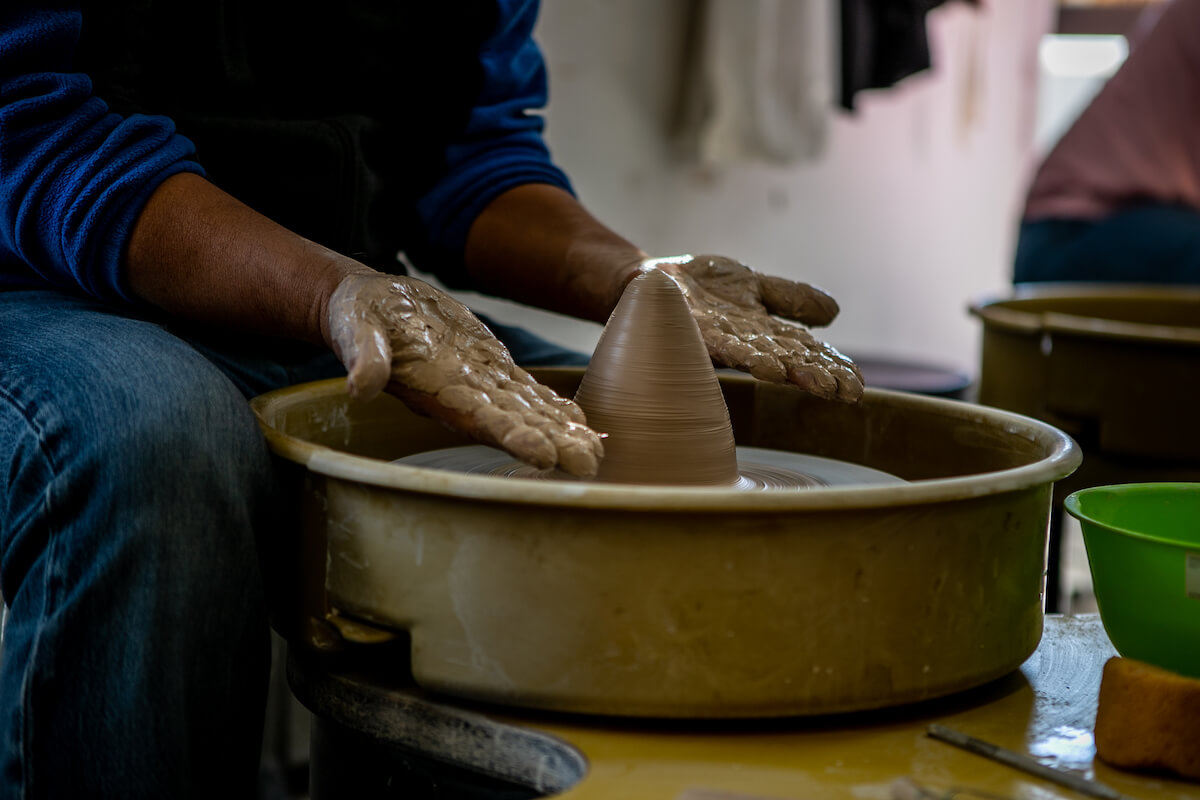This photo captures a moment in a pottery-making workstation where a man, only partially visible, is deeply engrossed in his craft. He is of a darker complexion, suggesting a different ethnicity from white. Seated and attired in a long-sleeve blue shirt and blue jeans, he focuses intently on his task. The image prominently shows his arms, hands, and legs, with his hands lifted and palms exposed, both covered in almost white, wet clay. In front of him is a round metal or steel wheel, likely a pottery spindle, on which a cone-shaped or triangle-like cylinder of wet clay is taking form. A green cup, possibly used for holding liquid, sits nearby. The blurred presence of another individual hints at a shared working environment, further emphasizing the collaborative nature of this meticulous and tactile craft.